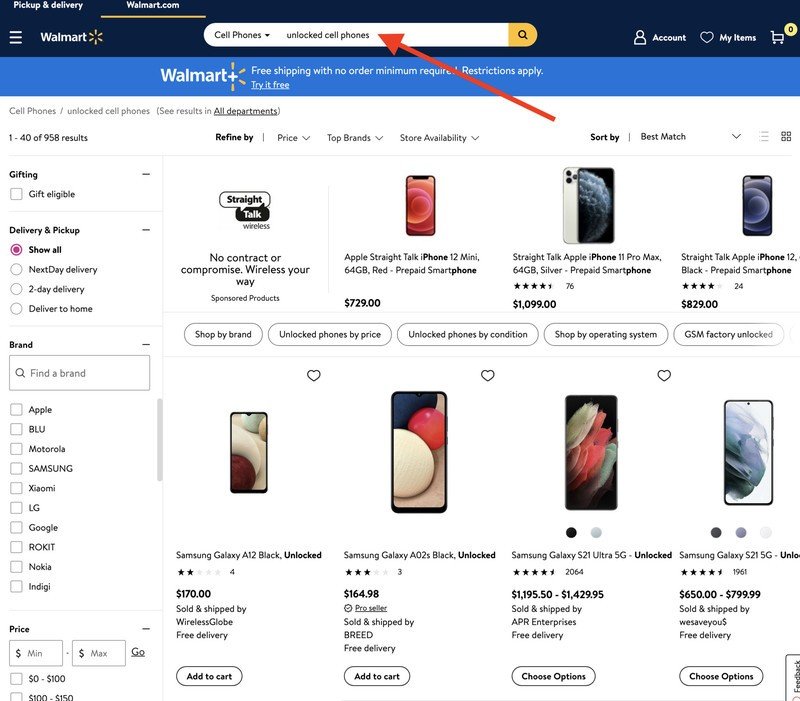This is a detailed screenshot of the Walmart app or webpage focused on a search for unlocked cell phones. The interface features a dark navy blue header with white text. On the left side of the header, there are two selectable options: "Pickup & Delivery" and "Walmart.com," with the latter highlighted by a yellow underline indicating it is currently selected. Flanking these options is the iconic Walmart logo. 

To the far left corner, a familiar hamburger menu icon with three stacked lines is visible. The center of the header boasts a prominent search bar, inside which is the text "unlock cell phones" with a red arrow pointing towards it, suggesting an active search query. To the right of the search bar, several key account management icons are displayed, including "Account," "My Items," and "Cart," all in white.

Immediately below the header is a sky-blue, centrally-aligned text banner promoting "Free shipping with no minimum order required. Restrictions apply. Try it free." The main body of the webpage is white, showcasing search results for cell phones. To the left, a vertical menu indicates there are "140 of 958 results," with options to refine the search by gift giving, delivery and pickup methods, and brand filters such as Apple, Samsung, and Google. Price filtering options are located at the bottom of this column.

The search results display two rows of cell phones, each row featuring four phones separated by gray borders. The top row consists of iPhones, while the second row displays Samsung Galaxy phones, complete with corresponding images, pricing, and brief descriptions.